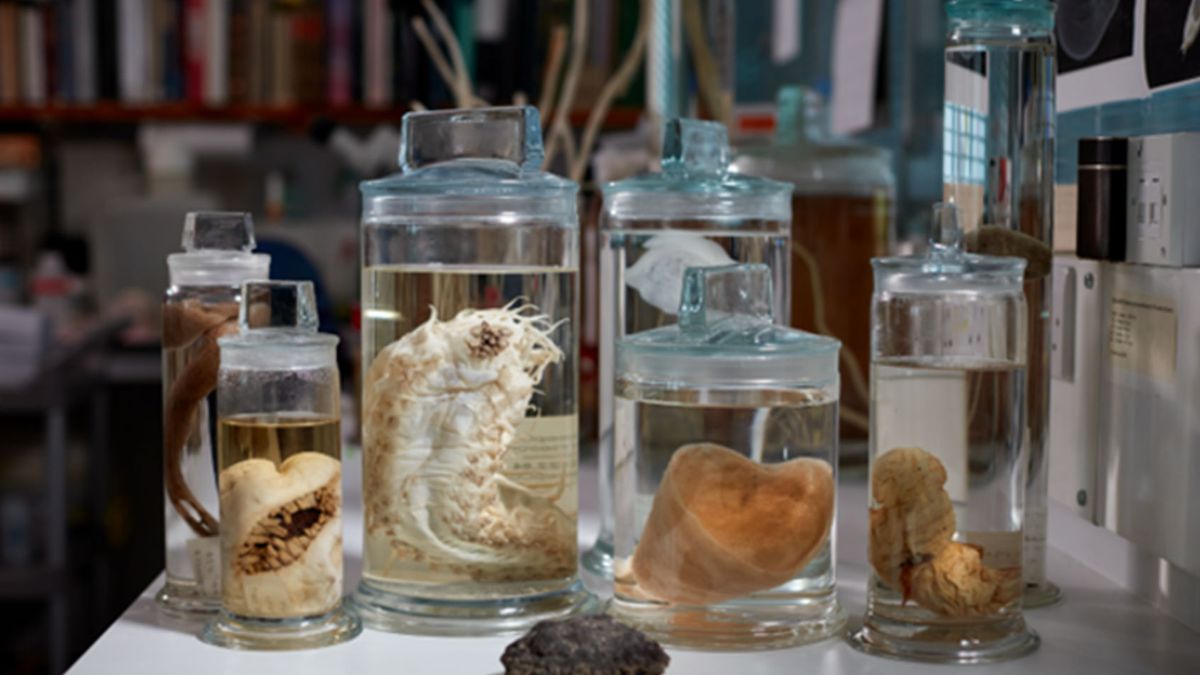The photograph, captured in a landscape layout, showcases a scientific setting, likely a lab or classroom. At the center of focus, a white table holds seven clear glass jars of varying sizes, each containing preserved scientific specimens such as insects, sea creatures, or other animal body parts. The jars are neatly arranged, with the front-most holding a large black rock. From left to right, the specimens inside the jars range in color from brown, off-white, white, pink to a brownish-tan hue. Some jars' contents are obscured, while others are clearly visible. The backdrop features a blurred array of shelves stacked with books, a white cabinet, and other indistinct laboratory equipment, all contributing to the authentic scientific ambiance of the room.